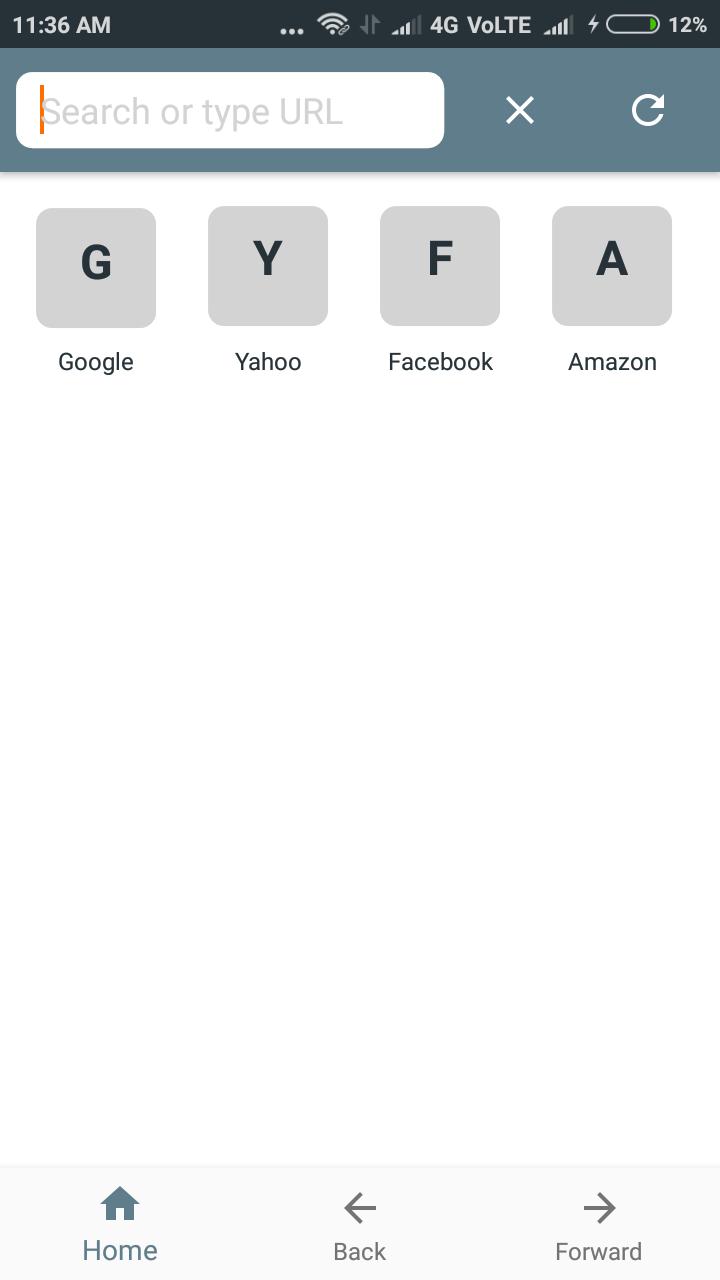The image is a vertically rectangular screenshot taken from a cell phone. The top section of the frame features a dark bluish-gray horizontal bar with white text and icons. On the left, it displays the time, "11:36 AM," while the right side shows various signal and Wi-Fi indicators along with a battery icon indicating 12% charge. 

Below this is a slate blue bar containing a white search or URL input field. Underneath this bar, there are four gray square icons arranged side-by-side, each with a single letter: "G" for Google, "Y" for Yahoo, "F" for Facebook, and "A" for Amazon. Beneath each icon is the corresponding name of the service. 

The background of the majority of the screen is a clean, white space. At the bottom, there's a very light gray horizontal strip containing navigation buttons for Home, Back, and Forward.